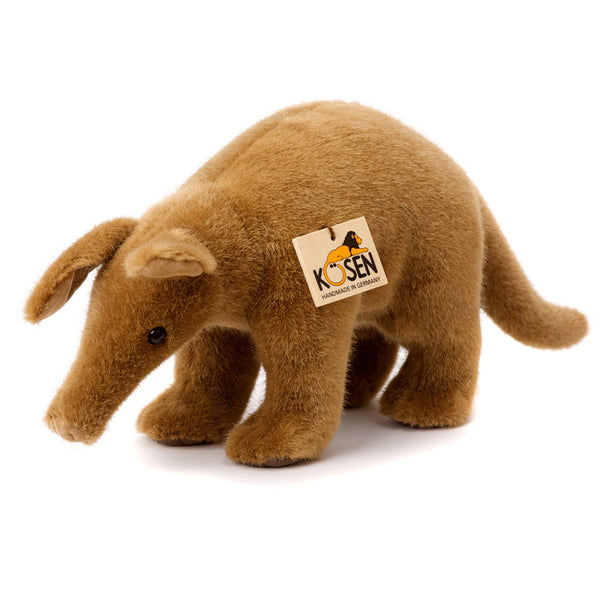This image features a highly detailed stuffed anteater with overall tan-brown fur. Its head, which sports a distinctive long snout characteristic of anteaters, is oriented toward the bottom left of the image. The anteater has black beady eyes and floppy ears. It is depicted standing, with its body and head facing left, and its long tail extending to the right side of the photograph. A notable feature is a white tag attached to the toy, prominently displaying the brand name "Kosen" (K-O-S-E-N) in capital letters. The 'O' in "Kosen" is creatively depicted as a curled lion's tail, with the lion lounging on top of the lettering. Below this, the tag reads "handmade in Germany," indicating the high-quality craftsmanship of this plush toy. The overall impression is one of soft texture and meticulous detail, suggesting it is a premium, handcrafted item.